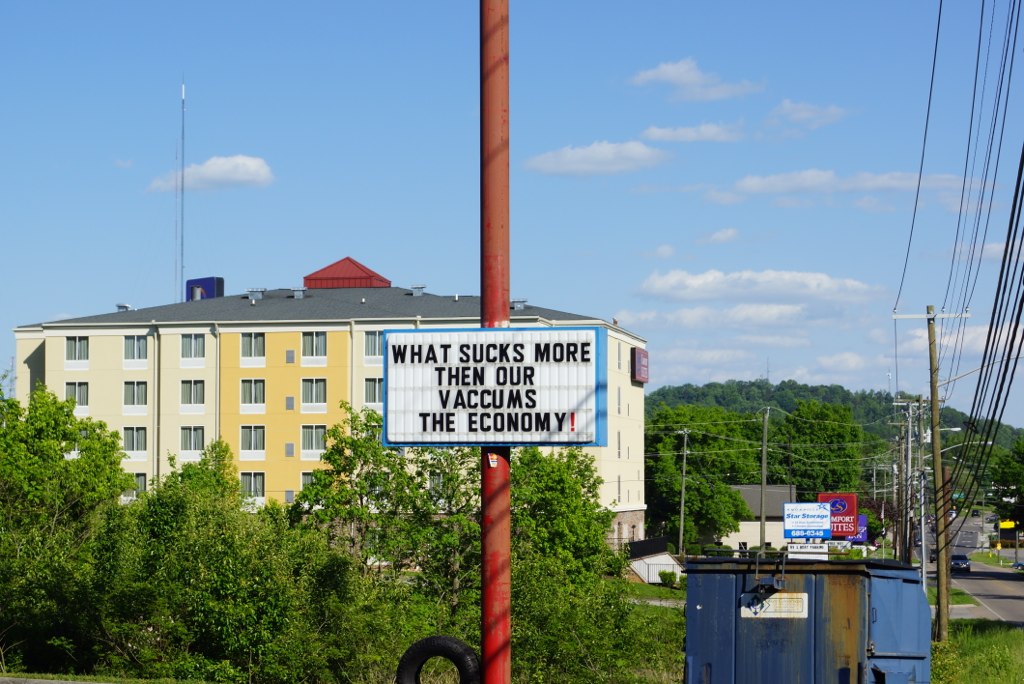This is an outdoor photograph featuring a tall hotel with an A-frame roof, standing out under a blue sky dotted with several clouds. The hotel's facade displays a mix of cream, tan, and golden-yellow hues. In front of it, a line of small trees and bushes runs parallel to the building, while behind the hotel, larger trees can be seen on a small incline, giving the impression of a mountainous backdrop.

Central to the image is a tall red metal pole with a white rectangular sign halfway up that reads, "What sucks more than our vacuums? The economy." The sign's text is black with a red exclamation point. At the base of the pole lies a car tire leaning against it. 

Directly in front of the camera is a blue, somewhat rusty dumpster. To the right of the dumpster, there's a road with power lines stretching above it, along which a few cars are traveling. Further down, the road is lined with additional buildings and business signs.